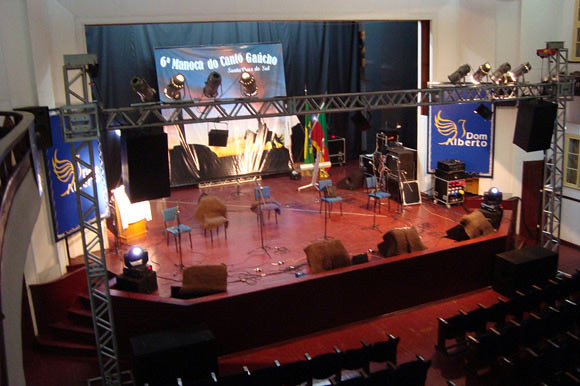The image captures a stage setup viewed from an upper balcony, likely on the second or third tier of an auditorium. The stage features a combination of seating options, including seven chairs arranged across the front; some are blue plastic while others are brown cushioned. Located between these chairs is an electronic amplifier. Flanking the stage on the left and right are aluminum-colored lighting structures rigged with additional lights aimed downward, illuminating the stage.

A red floor stretches across both the stage and the level ground of the lower auditorium, where all the connected seats appear to be flipped up. Access to the stage is provided via a set of stairs on the left side. The backdrop features a large blue curtain behind a screen displaying partially legible text. Additional posters bookend the stage, and among the decorations is noticeable wording in white against a blue background, including "D.O.M." and "Alberto" beneath a yellowish image of a bird—a dove. 

The lower perimeter of the stage hosts several electronic amplifiers facing the previously mentioned chairs, indicating the setup is likely for a musical performance. The overall scene is framed by a small border wall at the front, with a zigzagging metal bar structure connected to vertical beams that traverse the sides of the stage. There are also several visible speakers and a series of microphone stands positioned in front of each chair.